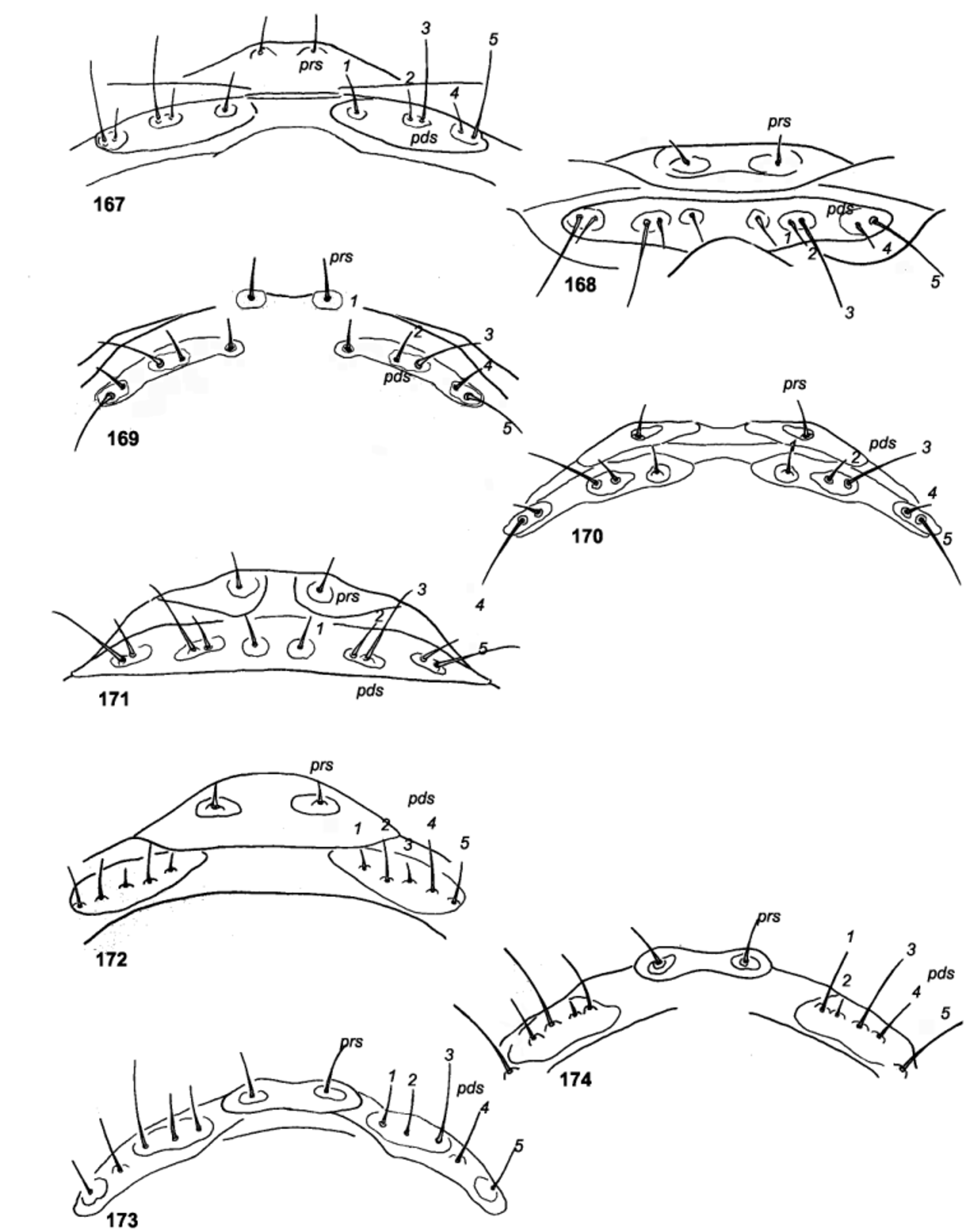The image presents eight black-and-white diagrams of various structures or shapes, each corresponding to an unidentified item. These diagrams are organized into two columns, with the left column featuring five structures labeled as 1067, 1069, 1071, 1072, and 1073 from top to bottom, and the right column showing three structures labeled 1068, 1070, and 1074. Each diagram exhibits intricate and irregular line patterns, along with circular outlines containing black hair-like projections. Each hair is individually numbered, and some are designated with the labels PRS and PDS, though their meanings are not provided. The structures resemble interconnected ovals, circles, and curved lines, hinting at a possible biological context, such as hair follicles or an insect anatomy, though the exact nature remains unspecified. The drawings lack any descriptive text, providing only numerical and lettered annotations.